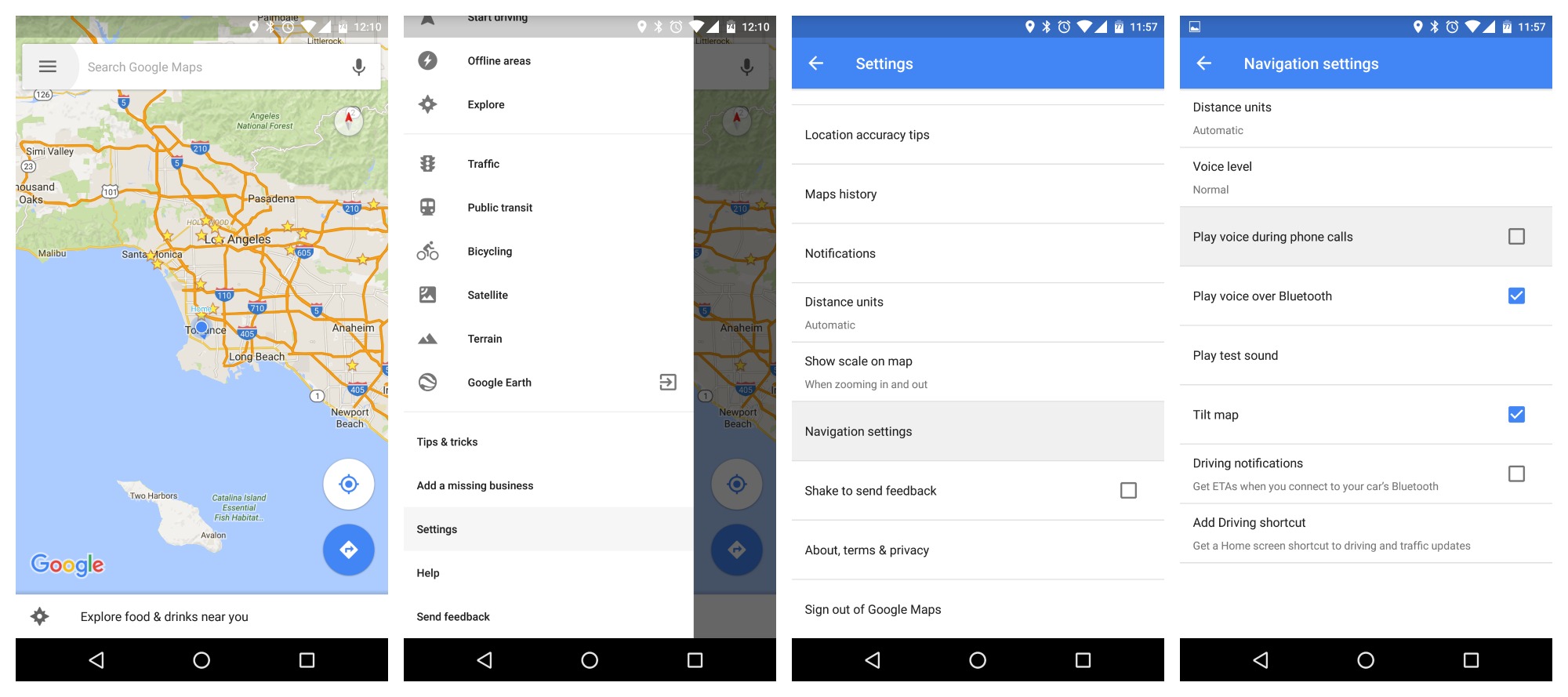The image depicts a series of four sequential screenshots, each capturing different user interface elements of a mapping application.

1. **First Screenshot**: Displays the main interface of a map application. In the top left corner, there is a hamburger icon (three horizontal lines), a search box to the right, and a microphone icon for voice search. At the bottom of the screenshot, there are control buttons: a left arrow, a circle, and a square.

2. **Second Screenshot**: Showcases the options menu, revealing various features you can explore within the app. The items listed include office areas, explore, traffic, public transit, banking locations, bicycling routes, SafeMe (a possible safety feature), trends, Google Earth integration, tips and tricks, a referring bonus, settings, help, and a send feedback option.

3. **Third Screenshot**: Focuses on the settings menu. Within this menu, items listed are location accuracy tips, map history, notifications settings, distance units (measurement preferences), an option to show scale on the map, and navigation settings which are highlighted in gray. Another feature mentioned is "shake to send feedback."

4. **Fourth Screenshot**: Identical to the content of the first three screenshots, it further emphasizes the presence of various interactive elements in the mapping application's user interface, ensuring seamless navigation and user customization options.